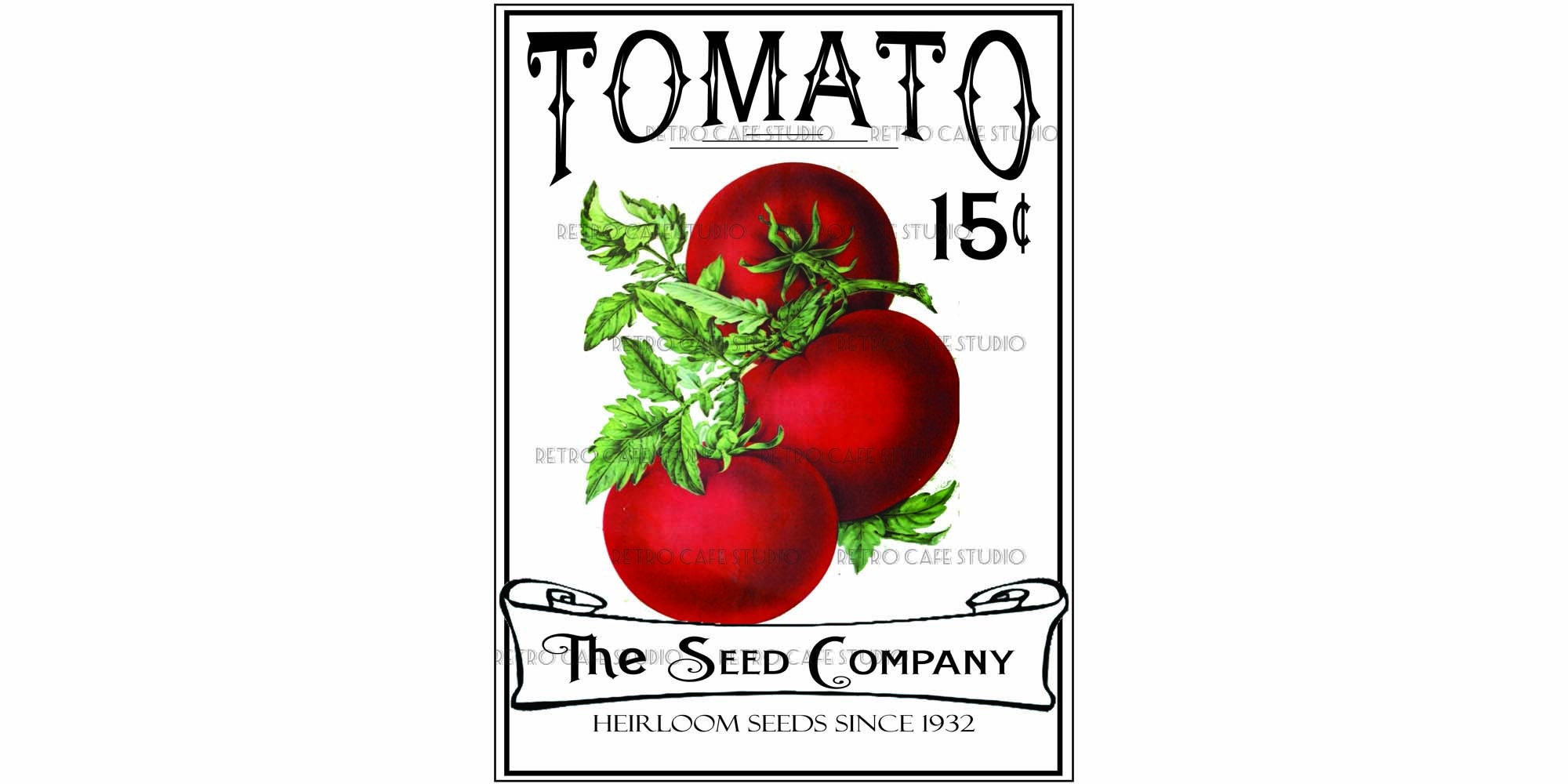This image illustrates a vintage seed packet that captures the essence of early 20th-century agricultural advertising. The packet is primarily white with a black outlined border. Dominating the top section, in an elegant arched black font, is the word "Tomato," with the price "15 cents" listed just beneath the final "O." Central to the design are three vividly ruby-red, plump tomatoes still attached to their lush, green vine, positioned such that one faces upward prominently displaying its stem, while the other two lie sideways. Each tomato is carefully depicted with light highlights, adding a sense of freshness and ripeness. Below the tomatoes, a meticulously hand-drawn black and white banner displays the text: "The Seed Company," with its script letters featuring more elaborate detailing on the initial capitals T, S, and C. Just underneath, in capitalized block letters, it proudly reads: "Heirloom Seeds Since 1932." The background of the packet includes some faded, watermark-like text, whose details remain subtle and difficult to decipher, adding an aged, nostalgic charm to the overall design.